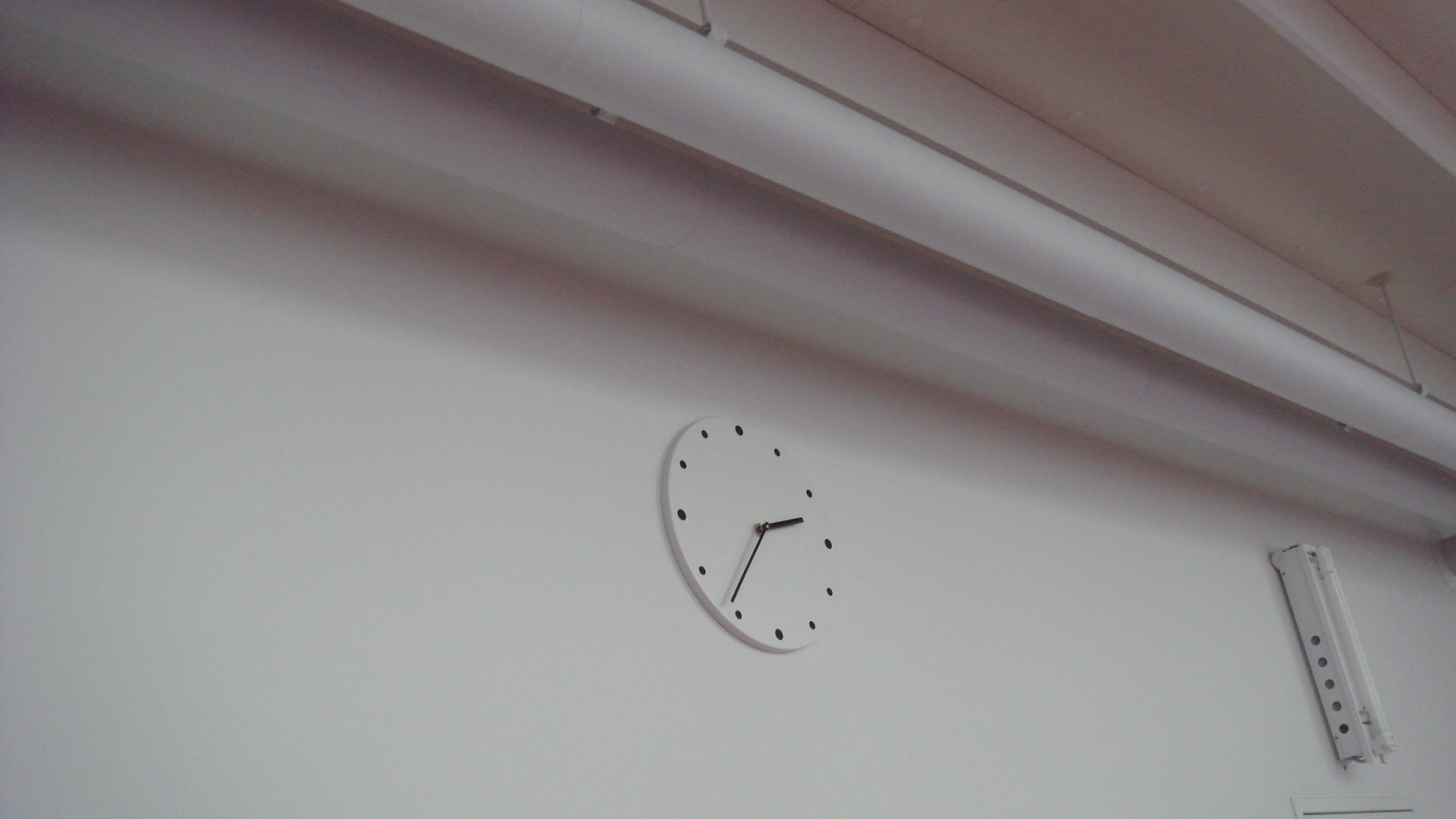This photograph portrays a minimalistic scene dominated by stark white tones. The focal point is a round, borderless school clock, standing out with its black color and dot markings for hours. The shorthand rests just past the 2 dot, while the longhand points around the 36 or 37 mark, indicating a time close to 2:37. Absence of minute markers and second hand adds to the simplicity and ambiguity of the clock. The white wall backdrop extends to the ceiling, where white-painted pipes are visible, indicating an industrial setting. On the right side of the frame, partially obscured, is an unidentified metal object, adding a subtle layer of intrigue to the otherwise bare composition. The photo is taken from an angled perspective, enhancing the depth and stark contrast of the scene.